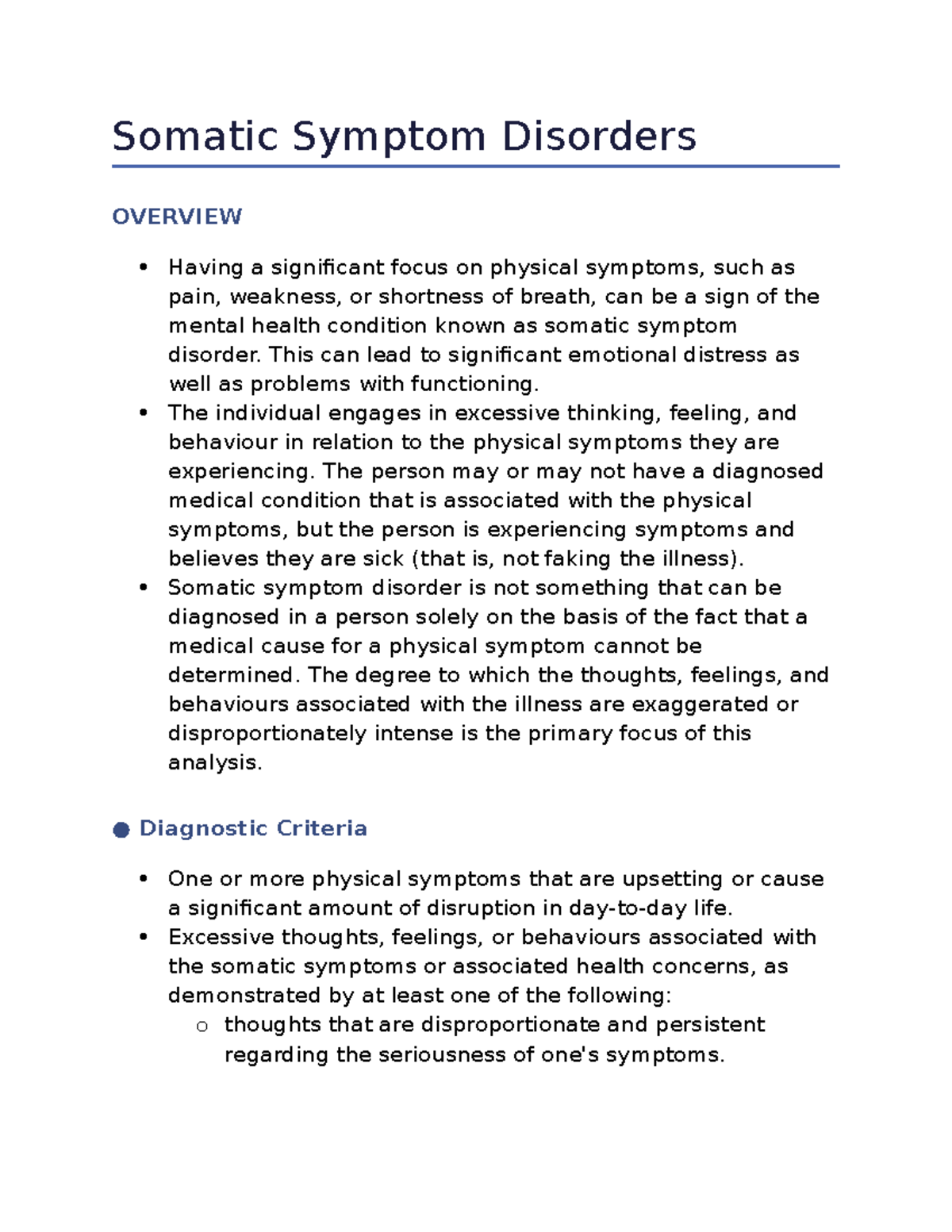The image contains an informative overview of Somatic Symptom Disorder, presented in a structured format with color-coded headers and bullet points for clarity.

At the top of the image, the title "Somatic Symptom Disorder" is displayed in bold black text, with each word capitalized. Below the title, there is an overview section with three key bullet points, all in black text. 

1. **Bullet Point One**:
   - Describes a significant preoccupation with physical symptoms such as pain, weakness, or shortness of breath, which may indicate a mental health condition known as Somatic Symptom Disorder.
   - Explains that this focus can result in considerable emotional distress and functional impairment.

2. **Bullet Point Two**:
   - Details how individuals with this disorder exhibit excessive thoughts, feelings, and behaviors related to their physical symptoms.
   - Clarifies that the presence of physical symptoms is perceived as genuine by the individual, regardless of whether a medical condition is diagnosed.

3. **Bullet Point Three**:
   - Emphasizes that Somatic Symptom Disorder is not diagnosed solely based on the absence of a medical explanation for physical symptoms.
   - Notes that the analysis focuses on the extent to which the person's thoughts, feelings, and behaviors are exaggerated or disproportionate.

Below this overview, there is a blue header titled "Diagnostic Criteria" in blue text. Under this header are two primary bullet points relevant to diagnosis:

1. **Diagnostic Bullet Point One**:
   - Specifies that the individual must experience one or more physical symptoms that cause significant distress or disrupt daily life.

2. **Diagnostic Bullet Point Two**:
   - States that excessive thoughts, feelings, and behaviors related to the somatic symptoms or health concerns must be present. This is further broken down into a sub-bullet point in white text:
     - Excessive thoughts characterized by persistent and disproportionate seriousness about one's symptoms.

This image serves as an educational and detailed guide to understanding the fundamental aspects and diagnostic criteria of Somatic Symptom Disorder.